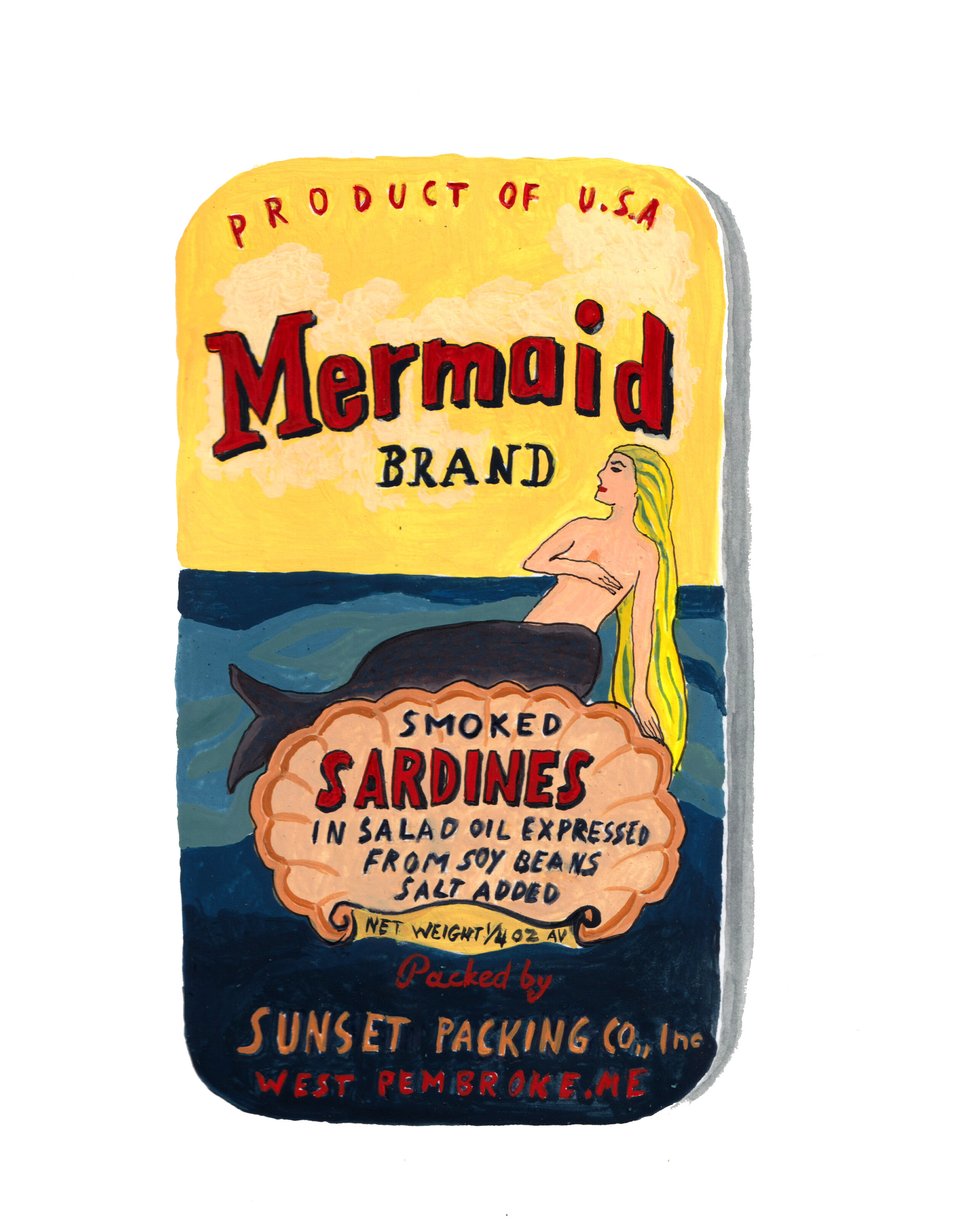The image exhibits a retro-style painting mimicking a sardine can, characterized by a distinctive three-dimensional gray edge curving behind the main depiction. At the top, in vintage rust-colored letters, it states "Product of USA." Below it, in bold, larger letters, it reads "MERMAID," followed by "BRAND" in all caps black letters. Central to the artwork is a detailed sketch of a topless mermaid with long blonde hair, red lips, and dark gray fish legs and fin. She sits on a clam shell, modestly covering her breasts with her right hand. 

The clam shell bears the inscription: "Smoked sardines in salad oil expressed from soybeans, salt added," and specifies the net weight as "one quarter of an ounce." Additional text, prominently in red, reads "Packed by Sunset Packing Company and Corporation, West Pembroke, Maine," enhancing the vintage packaging aesthetic. The mermaid's hair cascades down into the water, depicted with two shades of blue, contributing to the overall nostalgic and detailed artistic presentation.